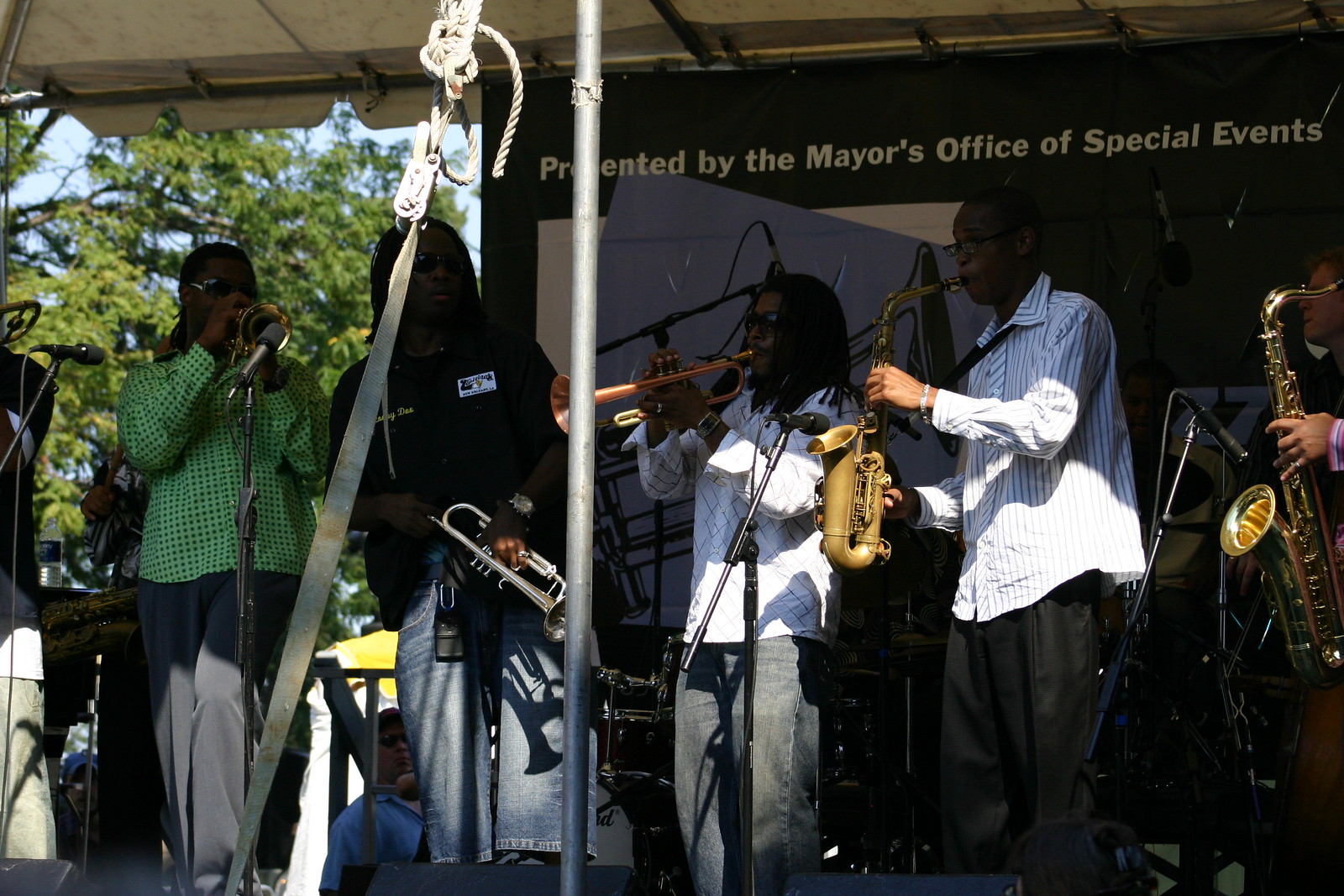The photograph captures a lively outdoor musical performance on a bright, sunny day, likely at a local summer music festival. It shows a band of at least six African American musicians, all seemingly wearing glasses or sunglasses, performing under a large white tent. The backdrop bears the text "Presented by the Mayor's Office of Special Events," suggesting this may be a city-sponsored jazz or blues festival.

From left to right on the stage, the musicians are:

1. A man in a green shirt and gray pants playing a trumpet, which has a copper finish.
2. A man with long braided hair wearing a black T-shirt and jeans, also playing a trumpet, but his instrument is silver.
3. Another person in a long white sleeve shirt and jeans holding a brass-colored trumpet.
4. A person in a white and blue striped shirt playing what appears to be an alto saxophone.
5. Cropped out towards the far right, another person can be seen holding a tenor saxophone.

The scene is set against a backdrop of green trees and a blue sky, indicating it’s a beautiful summer day. The performance is taking place in front of a decent-sized crowd, emphasizing a communal, festive atmosphere.